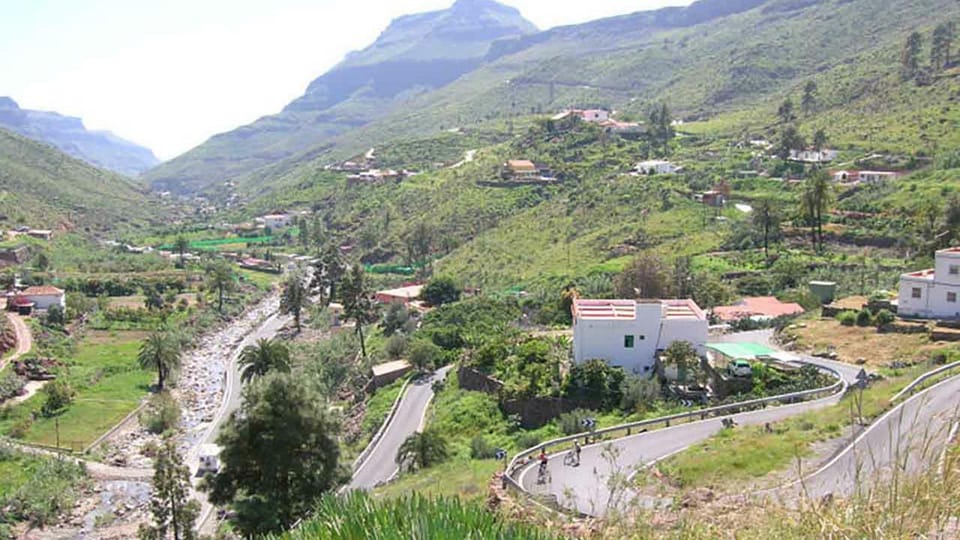This photo captures a serene mountain village nestled within a lush, green valley surrounded by rolling hills and towering mountain peaks. The perspective appears to be from atop a hill or a road, providing a head-on view of the quaint settlement. The winding, twisty roads, partly bordered by rocks or streams, snake through the idyllic landscape. Along one of these roads on the right, two small figures can be discerned riding bicycles, giving a sense of scale to the picture.

The village features a dozen or so small white buildings, many characterized by a cubic architecture, with some structures sporting reddish rooftops. The houses are scattered amidst abundant greenery and a variety of small trees, including several palm trees that lend a tropical feel to the scene. This verdant environment speaks to the lushness of the valley, suggesting a warm, perhaps tropical climate, which in turn hints that the location could be in Latin America or even a tropical part of Europe.

Overall, the image exudes tranquility and simplicity, depicting a quiet, residential village harmoniously integrated into the natural contours of the landscape, devoid of commercial buildings or heavy infrastructure.